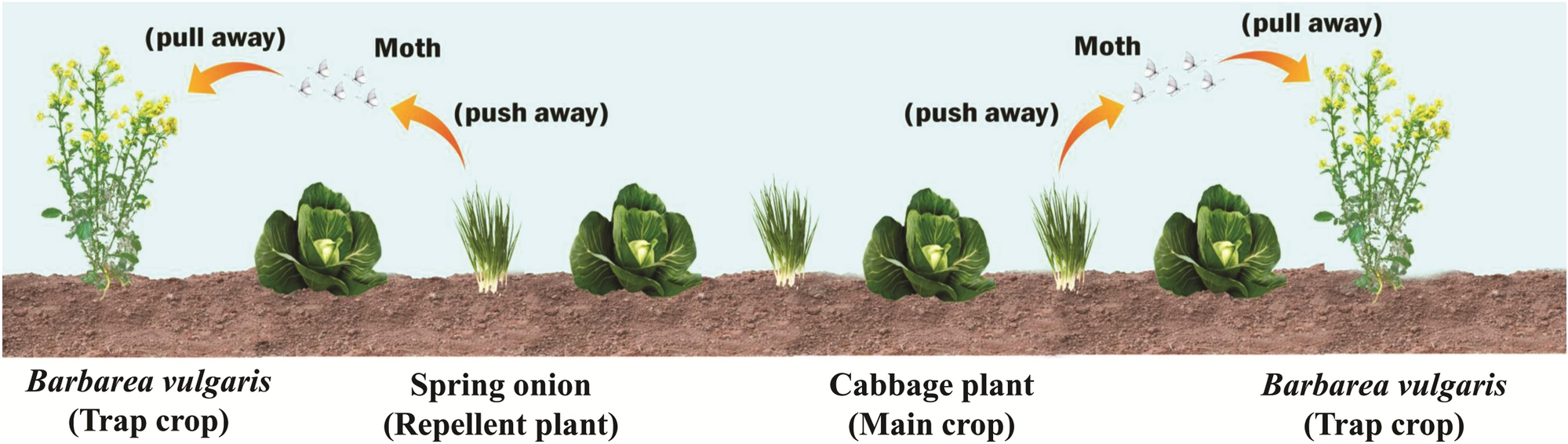This detailed image, seemingly excerpted from a biology textbook, depicts the interdependent life cycles of various plants, focusing on their roles in pest control and growth stages. The horizontally oriented photo showcases several crops rooted in soil, framed against a pale blue sky. From left to right, the image is labeled and features: *Barbarea vulgaris* (trap crop), spring onion (repellent plant), and cabbage (main crop), followed by another *Barbarea vulgaris* (trap crop). Orange arrows decorated with text such as "push away" and "pull away" are visible, pointing towards moths, illustrating the roles these plants play in pest management. The *Barbarea vulgaris* plants attract and trap moths, while the spring onions repel them, ensuring the cabbage plants can grow unhindered. The detailed diagram effectively outlines how these plants interact to secure each other's growth.